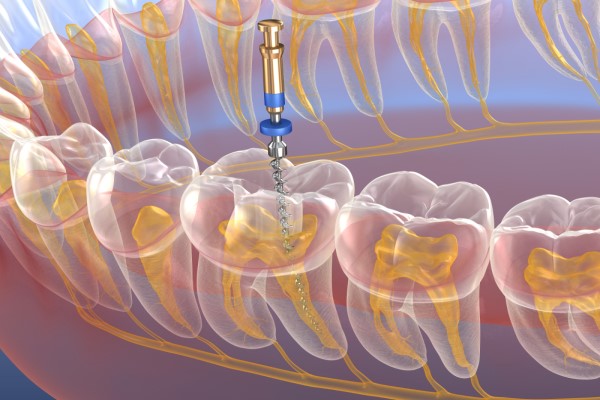This detailed illustration depicts a lower jaw with translucent teeth, revealing the dentin and nerves represented in gold. The image is similar to what might be found in a dentist's instructional textbook or used for educational purposes in a dental classroom. The teeth are arranged in a horseshoe shape, showing varying positions in the mouth. At the center, a blue and silver drill, tipped with gold, is seen penetrating one of the teeth, reaching into the roots, possibly demonstrating a dental procedure such as cavity filling or root canal treatment. The colorful and almost surreal appearance of the illustration gives it an unusual and slightly eerie vibe, reminiscent of a jellyfish with golden rings inside.